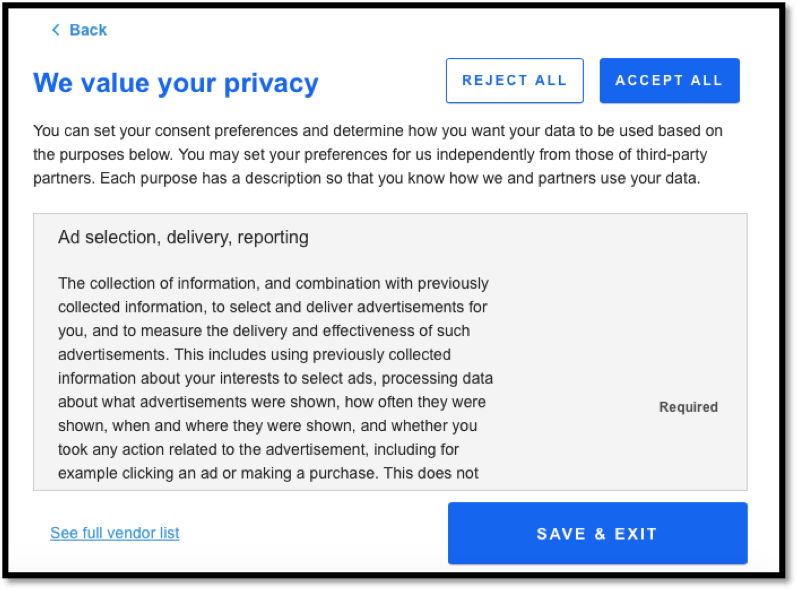This is a detailed screen capture from a website privacy settings page. The content is contained within a black box. At the top, in blue text, it reads, "We value your privacy." On the top right, there is a "Back" button. Below that are two buttons labeled "Reject All" and "Accept All."

Further down, in black text, the page states, "You can set your consent preferences and determine how you want your data to be used based on the purposes below. You may set your preferences for us independently from those of third-party partners. Each purpose has a description so that you know how we and partners use your data."

Following this, there is a section labeled "Ad Selection, Delivery, Reporting" which describes the collection of information and its combination with previously collected data to select and deliver advertisements for you, and to measure the delivery and effectiveness of such ads. This description includes details about using previously collected information about your interests to select ads, and processing data on what advertisements were shown, how frequently they were displayed, when and where they appeared, and whether you interacted with the ads, such as by clicking on them or making a purchase.

At the bottom, there is a blue button labeled "Save and Exit." To the right of this button, there is text that reads "See Full Vendor List."